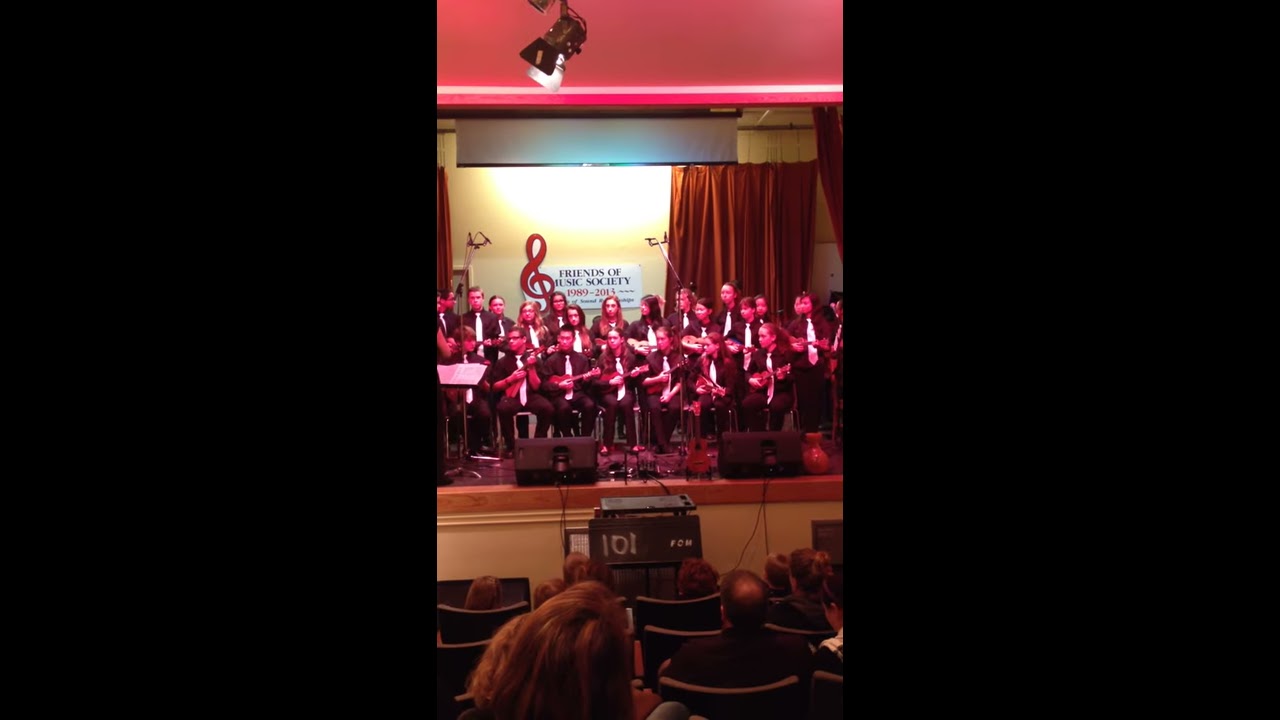The image depicts a stage performance by a school band, observed from the seats with the audience's backs facing us. The stage, illuminated by a red light, showcases around 30 male and female students, each dressed in black outfits paired with white ties. They appear to be holding white items uniformly with both hands, although these items do not resemble typical musical instruments and may be small guitars or ukuleles. The performance area features orange curtains pushed to the side, revealing a sign behind the band that reads "Friends of Music Society 1999 to 2014," decorated with a musical note. The front of the stage includes a podium, likely for a speaker, and is flanked by speakers distributed around the area. The audience seats are sparsely occupied, with individuals seated independently and scattered throughout.